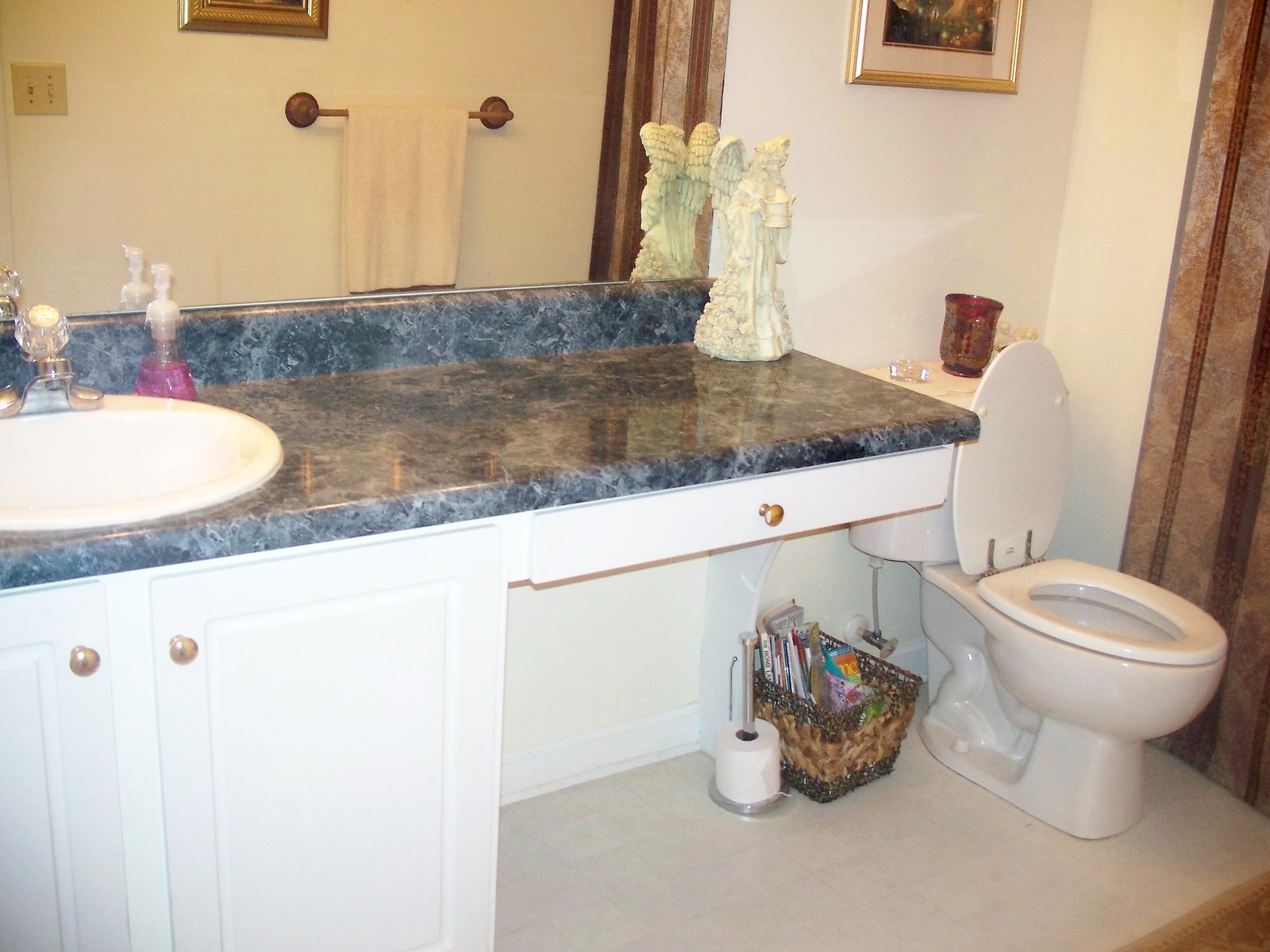The image depicts a cozy home bathroom with several distinct elements. On the far right, a brown and tan fabric decor lines the wall, providing a warm and rustic touch. Adjacent to this fabric, a white porcelain toilet sits neatly, accompanied by a pinkish-red candle holder and a clear glass item atop the toilet tank. Situated next to the toilet on the floor, a brown and metal rack holds an array of magazines, while a nearby metal paper towel holder dispenses toilet paper.

Above the toilet, a gold-framed painting hangs, although much of it is out of the frame, adding a touch of elegance. To the left of the toilet, white cabinetry with gold handles provides additional storage; it features a pull-out drawer and dual doors that open up. The vanity counter is made of chic bluish marble, which houses a detailed white porcelain angel statue and offers ample space.

A large mirror above the counter reflects the opposite side of the bathroom, revealing a brown towel rack adorned with a white towel and another gold-framed piece of art. The reflected image also shows the continuation of the marble theme, a useful light switch with dual controls, and the edge of the countertop.

On the marble counter surface, there is a white sink fitted with a silver faucet that has a clear plastic or crystal handle, exuding a modern feel. Next to the faucet, a purple pump soap dispenser adds a pop of color to the serene yet sophisticated design of the bathroom.